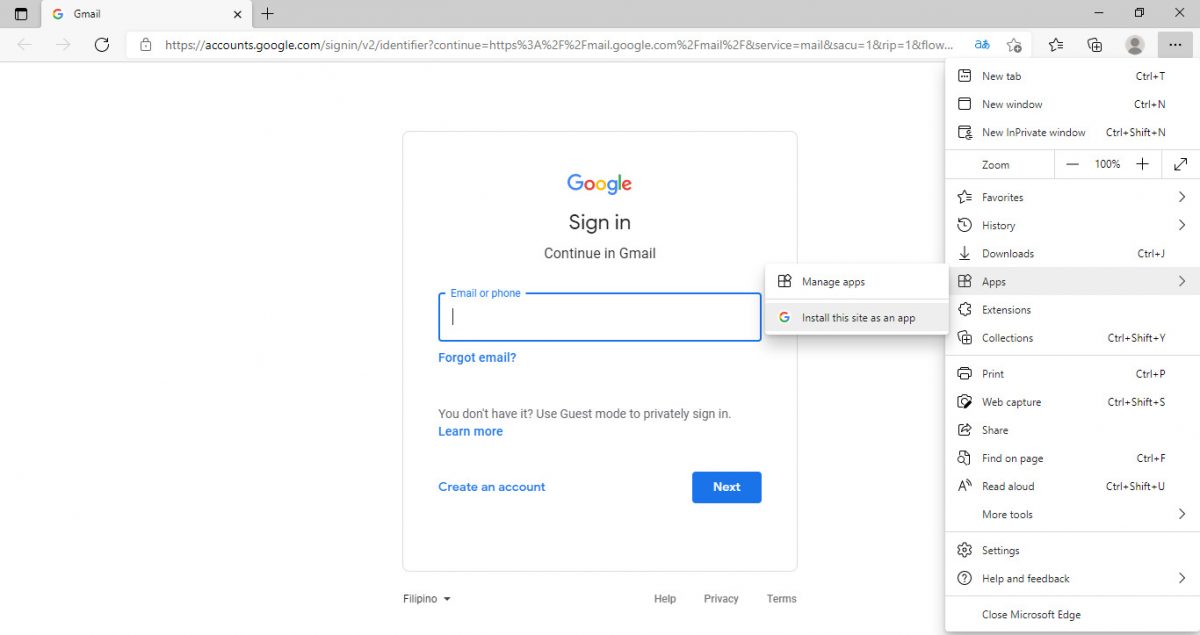This image captures a web browser interface displaying the sign-in page for "Googly," accessible via the URL "account.googly.com." The centerpiece of the page features the "Googly" logo, artfully rendered in four distinct colors: red, blue, yellow, and green. The headline reads "Googly Sign In," followed by a prompt to "Continue to Gmail." 

Beneath this, there's a text field labeled "Email or Phone," surrounded by a blue outline, with the input guidance text also appearing in blue. Below the text field, there is a link stating "Forgot email?" in blue font, positioned above a line of black text providing alternative sign-in options: "Don't have it? Use Guest mode to privately sign in. Learn more," with "Learn more" also highlighted in blue.

Towards the bottom of the sign-in panel, the user is given two options: on the bottom left, a link to "Create account," and on the bottom right, a blue "Next" button. Additionally, the bottom-left corner of the page features the language option "Filipino," whereas the bottom right lists three essential tabs: "Help," "Privacy," and "Terms."

The right-click context menu visible on the right side of the image offers options such as "Manage app," "Install this site as an app," and displays the browser's top navigation, showing "New Tab." The browser menu is extensive, featuring options like "New tab," "New window," "New InPrivate window," "Zoom," "Favorites," "History," "Download," "Apps," "Extensions," "Collection," "Print," "Web capture," "Share," "Find on page," "Read aloud," "More tools," "Settings," and "Help and feedback." At the very bottom of the context menu, there is an option to "Close Microsoft Edge," indicating that this is the browser in use.